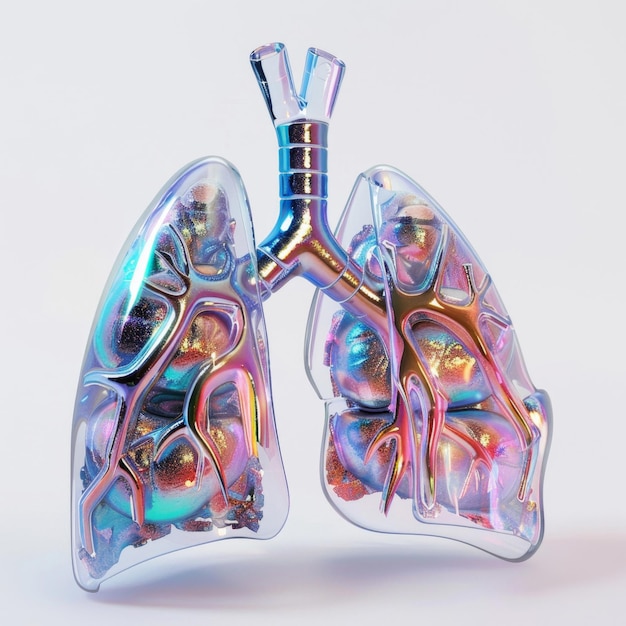The image features a detailed and striking model of a pair of lungs, prominently set against a gray background. The lungs appear transparent, crafted from what seems to be glass or see-through plastic, showcasing an intricate internal structure. The trachea and bronchi are clearly visible, leading into the multitude of vein-like bronchioles within each lung. There is a distinct mix of colors running through the tissues including pink, blue, orange, red, yellow, and purple. The tubes and pipes integrated into the lungs are designed with a shiny black metal, providing a stark contrast to the vibrant hues of the tissues. The left lung shell appears smoother, whereas the right one has a slight jut on one side, perhaps due to the angle of the view. Underneath the model is a subtle shadow, enhancing the three-dimensional effect against the white background.